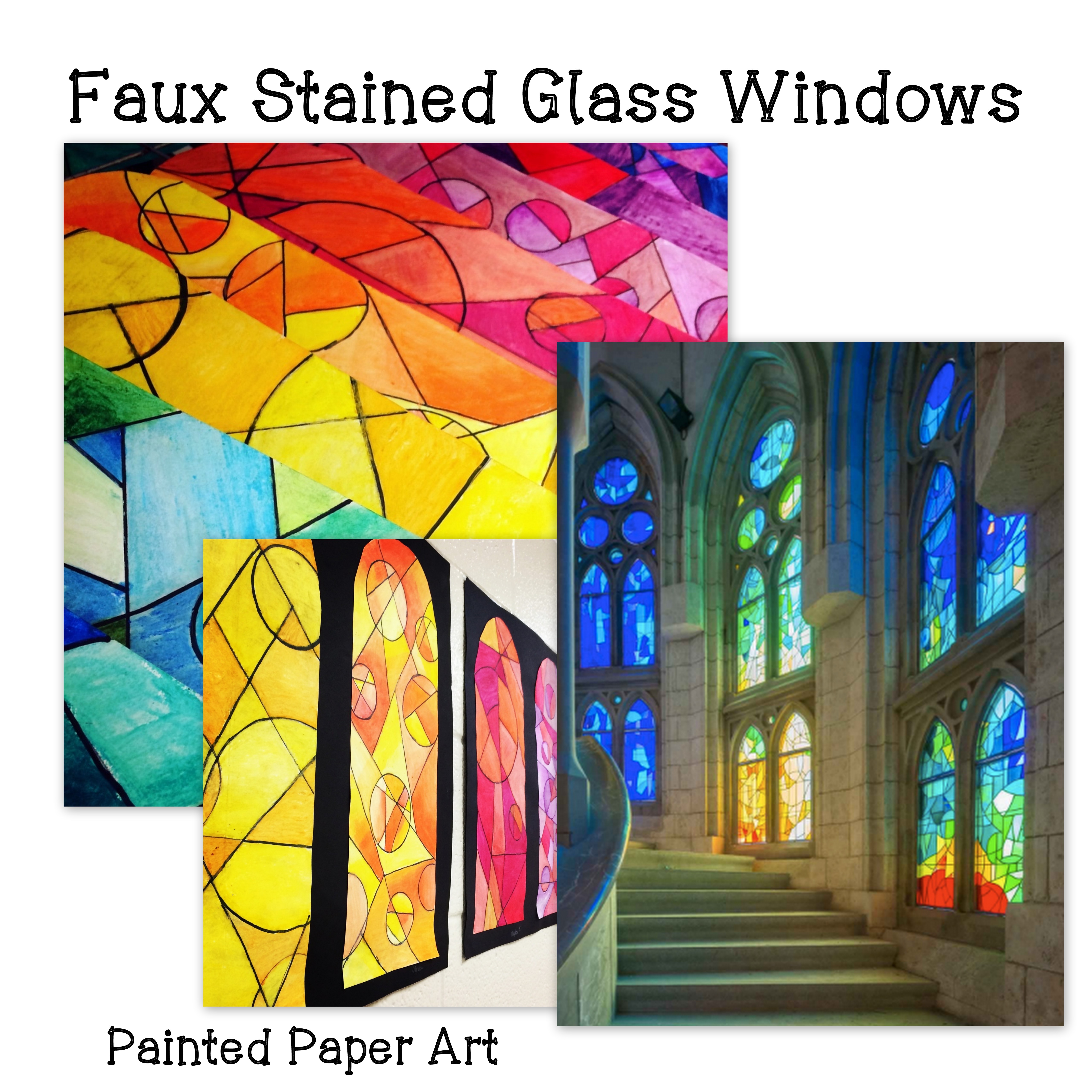The image is a digitally composed collage featuring elements that mimic stained glass art using paint and paper. It starts with black text at the top reading "Faux Stained Glass Windows" and similar black text at the bottom left that says "Painted Paper Art". The collage is set against a white background and presents three distinct segments. 

In the lower right corner, there's a realistic photograph depicting the interior of a church or cathedral, showcasing arched stained glass windows in vibrant colors of green, blue, and red along the right-hand wall, with a staircase curving up to the left. This scene exudes an air of solemnity and grandeur typical of such sacred spaces. 

To the upper left, there's an image that appears to be a series of stained glass windows rendered in colored pencil, creating a drawing-like effect that mimics the intricate designs of stained glass. This image gives the illusion of a hand-drawn depiction, emphasizing the artistic process.

Beneath this, the collage includes another smaller image showing framed mock-ups of stained glass windows. These are crafted from painted paper and hung up on a white wall, with various color schemes including green, yellow, white, and shades of blue, pink, and orange, highlighting the versatility of creating faux stained glass art. 

Together, these components combine to form a visually rich and detailed description of stained glass-inspired artistry, presented through different mediums and techniques.